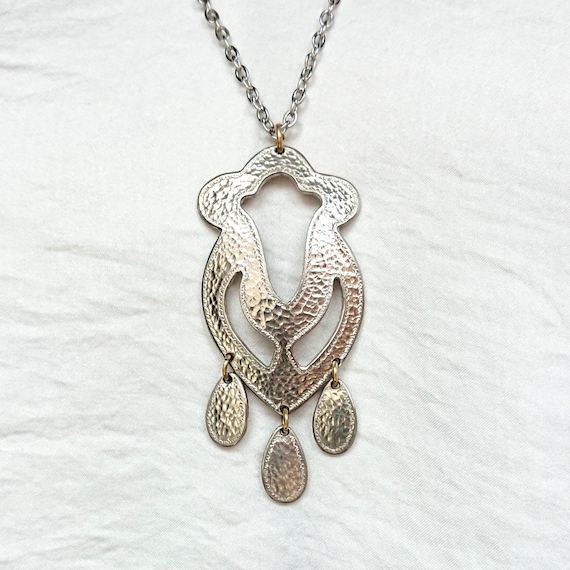This is a close-up photograph of a silver necklace with an ornate, uniquely-shaped pendant. The chain itself, which appears to be a simple metal chain, is partially visible and has a gold clasp. The pendant, attached to the chain, is an intricate design resembling a flower or an abstract acorn. The pendant's main body features a textured, shiny silver surface with a carved appearance, tapering toward a narrow base. The bottom edge of the pendant has three smaller, identical teardrop-shaped ovals dangling from it, giving the whole piece an elaborate and decorative look. This entire arrangement is laid on a white, slightly wrinkled background that could be a piece of linen, tissue paper, or a tablecloth, enhancing the pendant's reflective quality and detailed craftsmanship.